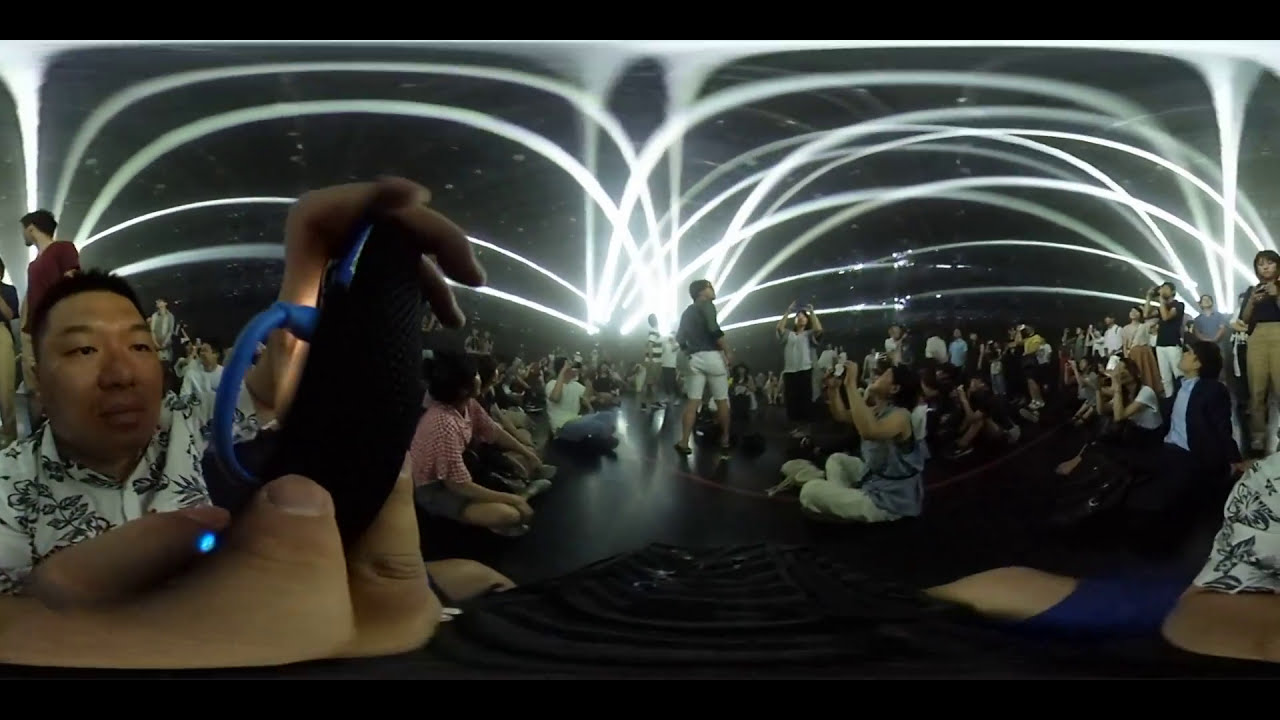This indoor image captures an event or concert bustling with activity. In a darkened room illuminated by rows of bright, white neon lights arching across the black ceiling, hundreds of attendees are seated cross-legged on the floor. Many of them, with dark hair and skin, are holding cameras and phones, capturing the moment. A man in a patterned white shirt with black designs is prominently featured in the close-up left corner, holding a dark phone connected to a blue cord, seemingly taking a photo. Nearby, a woman sits cross-legged on the floor, wearing a patterned shirt and white pants, aiming her camera toward the ceiling. In the distance, a man stands with his back to the camera, dressed in white shorts and a green top. The room is alive with the energy of countless people collectively gazing upward and documenting the experience under the glow of the striking neon lights.